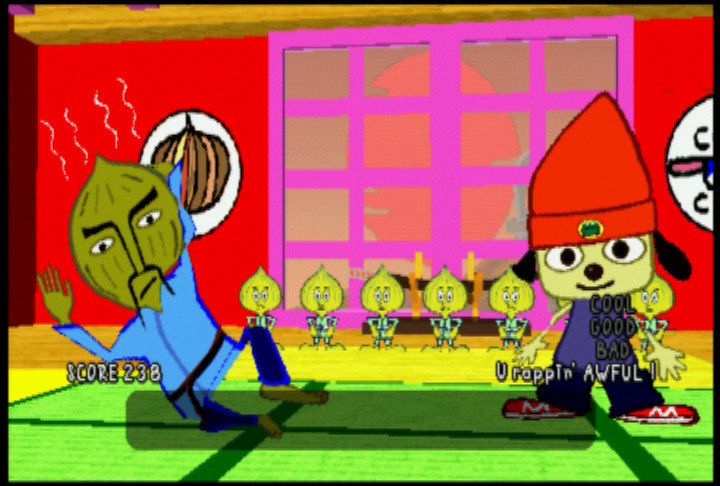This is a screenshot from a vibrant, cartoonish video game with bright colors and a nostalgic feel, reminiscent of old NES or handheld games. On the right side, a dog character stands on two feet, wearing a distinctive red beanie with a yellow logo, red shoes with an 'M' on them, blue pants, and a lighter blue shirt. On the left, an onion-faced man, who appears Asian with a Fu Manchu mustache, is dressed in a gi and slippers. The scene suggests a rap battle as words like "cool," "good," "bad," and "you rap in awful" are displayed. The setting features a green striped floor in the foreground and a yellow floor in the background, with a group of smaller onion-faced characters observing. A large, vivid red back wall houses a floor-to-ceiling pink window. Additional details include a clock partially visible next to the dog character and wooden paneling across the top of the wall. The score is shown in the lower right corner, contributing to the dynamic and entertaining atmosphere of the game.